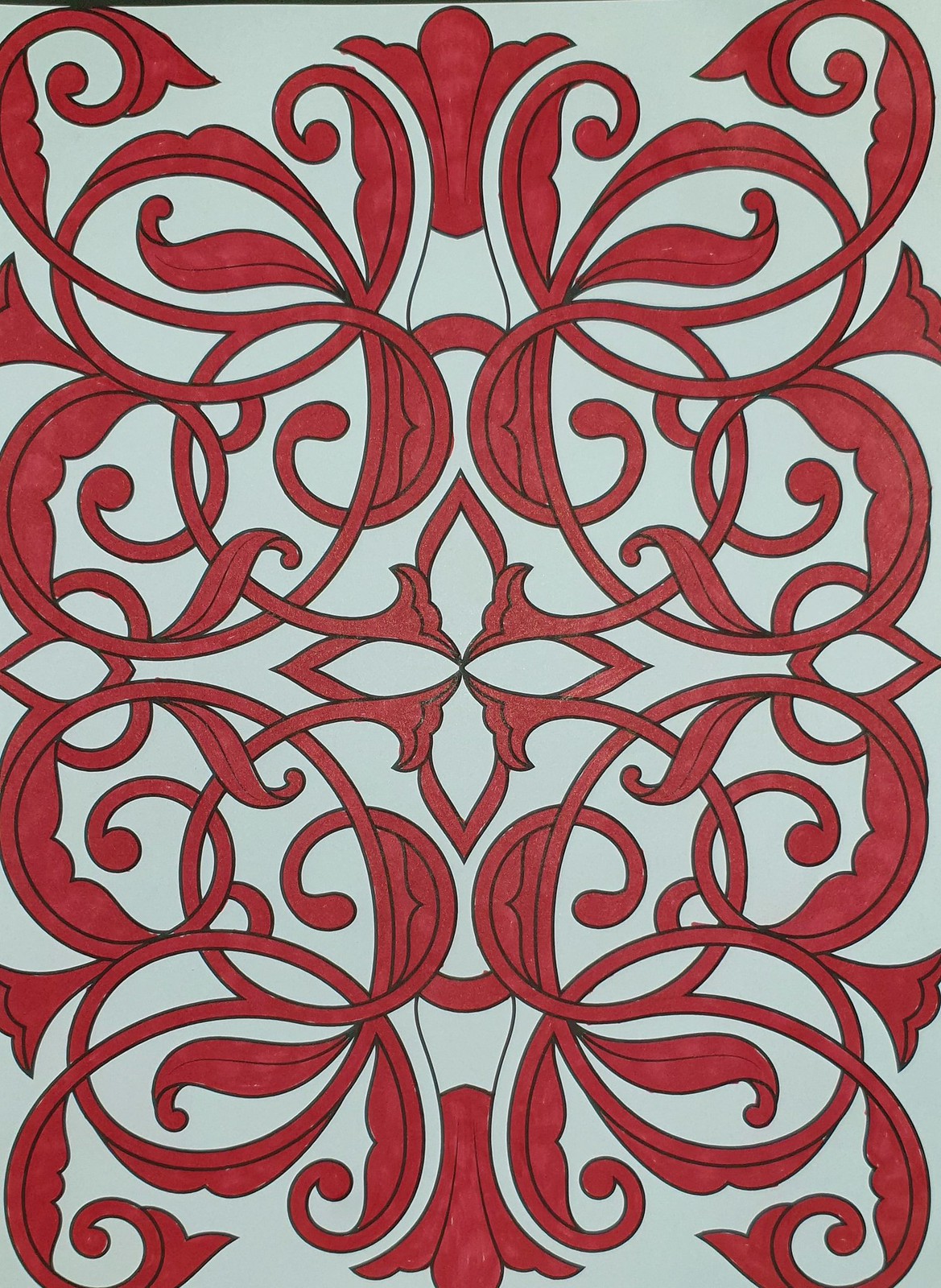The image features a striking and intricate logo set against a white background. The design is predominantly red and appears to be a modern take on vintage patterns, reminiscent of designs often seen on classic furniture. The logo is composed of an elaborate network of interwoven lines and circles that overlap to create a complex, almost floral motif. While it evokes a Paisley-like aesthetic, it distinctly maintains its unique character.

Central to the design is a prominent red flower that stands out amidst the surrounding pattern, acting as the focal point. The overall composition of the logo gives off a leafy impression, with the various elements converging harmoniously towards the center. The combination of circles, lines, and floral elements results in a visually engaging and richly detailed logo that marries both vintage and contemporary styles.